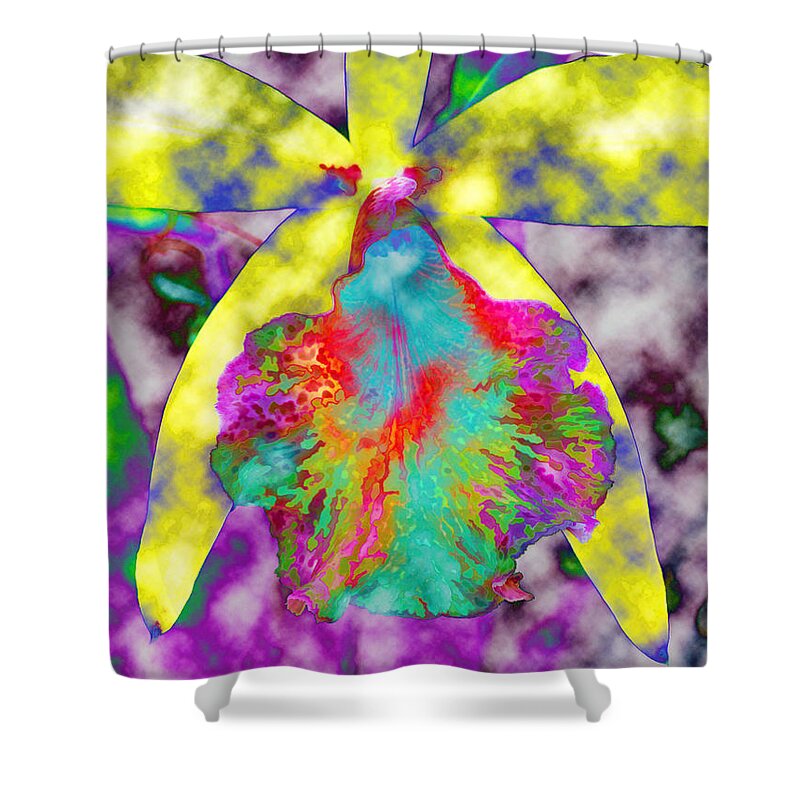The image features a decorative shower curtain set against a plain white background with no visible borders. The curtain is about 5 inches high and 4 to 5 inches wide. At the top, there's a long white bar that bows outward in the center, from which a dozen or so circular metal hooks are hanging. The shower curtain itself showcases an abstract design with a background predominantly in shades of purple, ranging from light to dark, with touches of green and blue.

Overlaying this background is a large, yellow shape resembling a marijuana leaf, outlined in blue, that extends off the top of the image. In front of this is a bold, colorful form that has the outline of a mushroom, rendered in a spectrum of red, pink, blue, green, and yellow hues. This form creates an explosion of color towards the center of the lower half of the image, with bright blue at the center, radiating outwards into red, yellow, green, and purple at the edges.

Beneath the shower curtain, the white feet of a clawfoot tub are visible, casting a small shadow between them, anchoring the whimsical, vibrant design in a traditional bathroom setting.